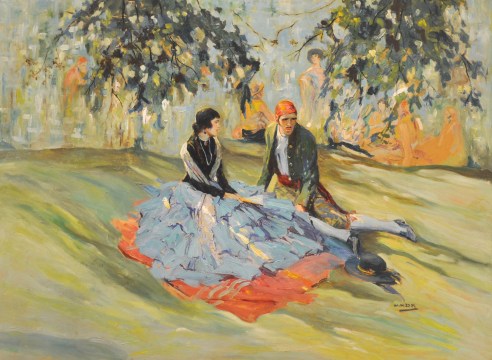The painting captures a tranquil scene set in a park, featuring a couple as its focal point. In the foreground, a young woman is elegantly draped in a large, eye-catching dress. The lower section of her dress is a vivid blue, while the upper portion showcases contrasting black and white tones. She is comfortably reclining on a bright red blanket spread on the lush grass. Beside her, a man dressed in what appears to be historical Spanish attire complements the scene. He sports a dress jacket and a crisp white shirt, accessorized with a distinctive ribbon-like scarf hanging from his waist. The couple appears to be deeply engaged in conversation, suggesting a romantic date. The background is populated with other park-goers, although they are rendered with less detail, emphasizing the couple's intimate moment as the central focus of the artwork.